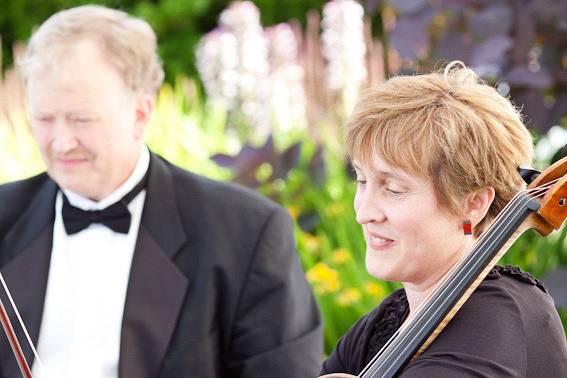This photograph, taken outdoors, features two people playing string instruments amidst a blurred background filled with colorful flowers, including white, purple, and yellow among green leaves and grass. On the right, a woman with short, wavy, reddish-blonde hair and a light complexion is visible from the chest up. She wears a dark black dress and bright red clip-on earrings. She holds a violin against her left shoulder, looking down and smiling at her instrument. On the left, an older man with light skin and thin, receding blond hair wears a black tuxedo, white shirt, and black bow tie. He too plays a string instrument. Their combined presence creates a harmonious blend, accented by the serene garden backdrop.